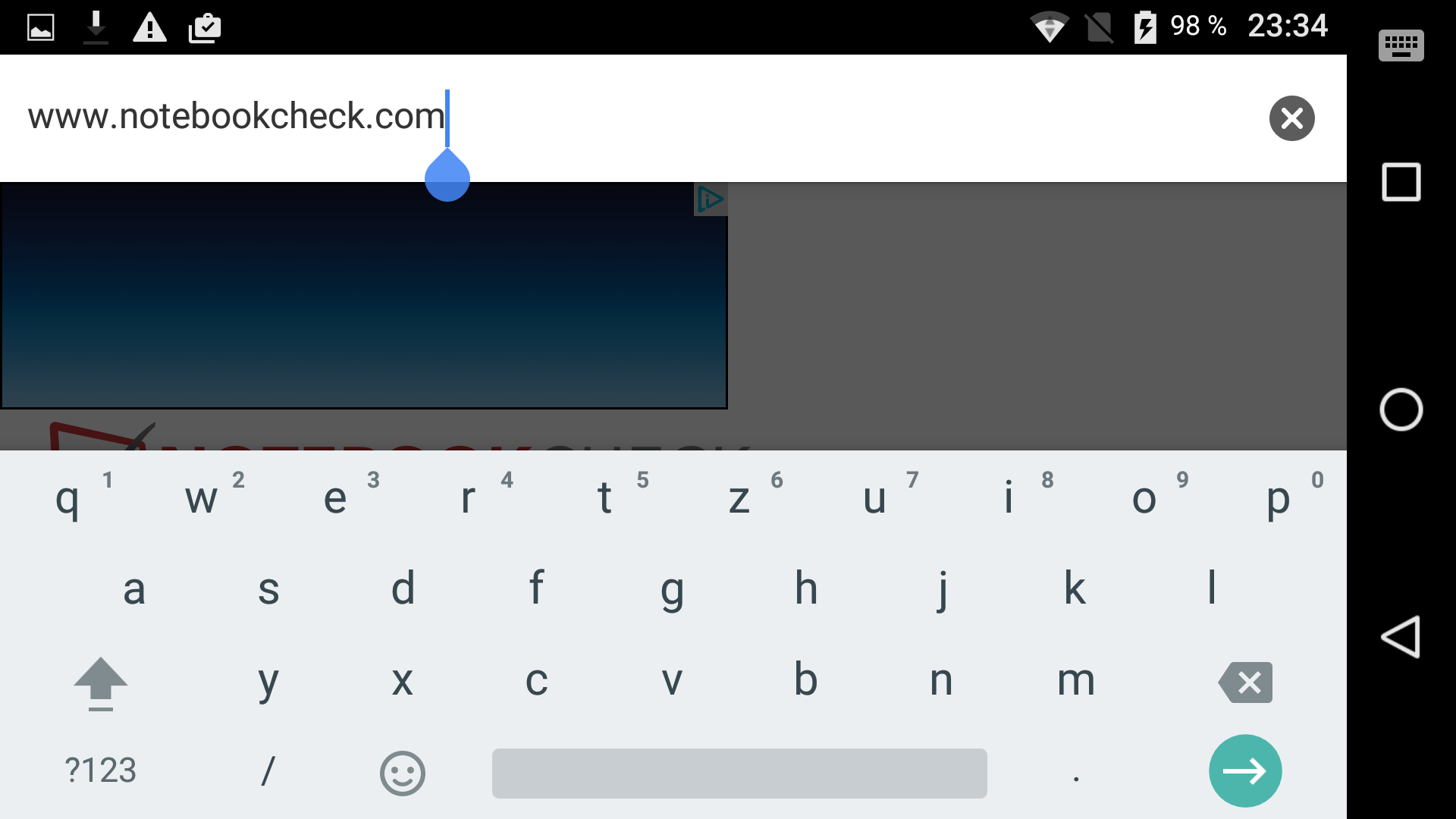This is a detailed screenshot from an Android phone, capturing various elements on the screen with precision. At the top bar, there are status icons including an image icon, a high-strength Wi-Fi signal, a battery charge of 98%, and the current time displayed as 23:34. Unique to this screenshot is the placement of the navigation buttons, which are conventionally at the bottom, but here they are positioned on the right side, a characteristic feature of an LG interface.

The screenshot prominently features a browser interface. Beside the URL box is a partial view of a site, notebookcheck.com, highlighted by a blue cursor, and there's an 'X' button for closing the page on the far right. Below the URL bar, the display shows a combination of blue and dark gray backgrounds within a square. The blue section is a solid color, while the dark gray area has a distinct red line just below the blue square.

The remainder of the image captures a QWERTY keyboard layout in lowercase mode. It includes functional keys such as shift, backspace, enter (in green), space bar, emoji selector, and a key for numbering and punctuation. The keys have black letters on a very light gray background, making them easily readable. The detailed depiction highlights the efficiency and design of the user interface on this particular Android device.